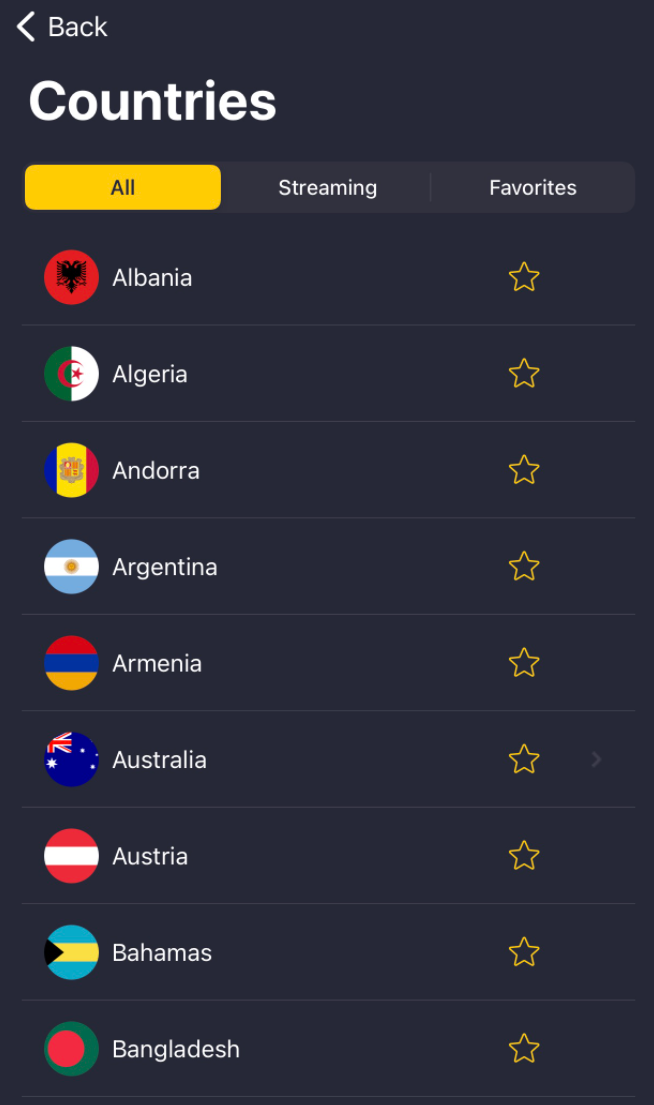The image features a sleek interface displayed on a black background. At the top left corner, an arrow accompanies the word "Back," positioned above the label "Countries." Just beneath, a yellow tab states "All," with "Streaming" and "Favorites" appearing to the right in white lettering on black background tabs. In the central section, a vibrant and colorful alphabetical list of countries is showcased, starting with Albania, Algeria, Andorra, Argentina, Armenia, Australia, Bahamas, and Bangladesh. Each country is represented by its respective logo on the left, and to the right of each name and logo, there are gold stars that are hollow in the center with golden edges. This visually rich interface presents a vivid and organized representation of the countries.